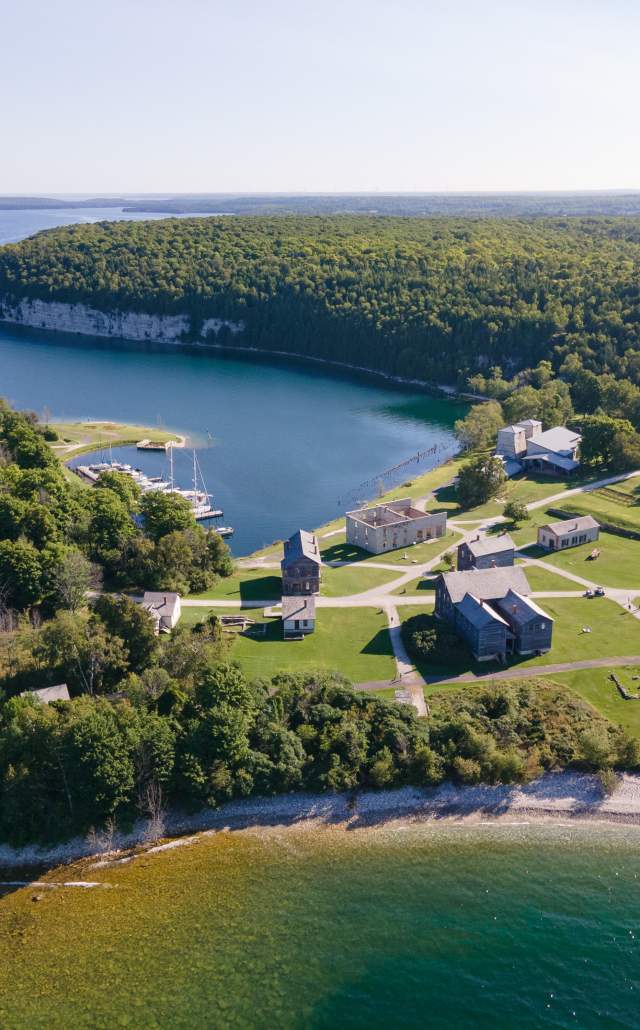This aerial photograph captures a picturesque small town nestled on a peninsula adjacent to a large lake. The town features an array of houses, ranging from quaint one-story cottages to larger two-story homes. Notably, one of the central buildings appears to be under construction, evident by its missing roof. The houses are neatly organized in squared patches of landscaped property, connected by a network of narrow, grey footpaths that crisscross through the area.

To the left side of the image, there is a dock with sailboats moored in a calm, turquoise-green bay. The serene waters transition to a lighter blue towards the bay's center, with the shorelines adorned by rocky beaches. Towards the top of the image, the peninsula curves around, sheltering the bay, and you can spot another small pool of water, likely a pond. 

Surrounding the bay and extending into the background, a dense forest envelopes the area, punctuated by a palisade-like rock formation on the upper left side. The expanse of trees creates a lush, green horizon, blending seamlessly into the hazy sky above. The foreground of the image also reveals a few cars parked near the houses and people walking along the streets, adding a lively touch to this scenic locale.